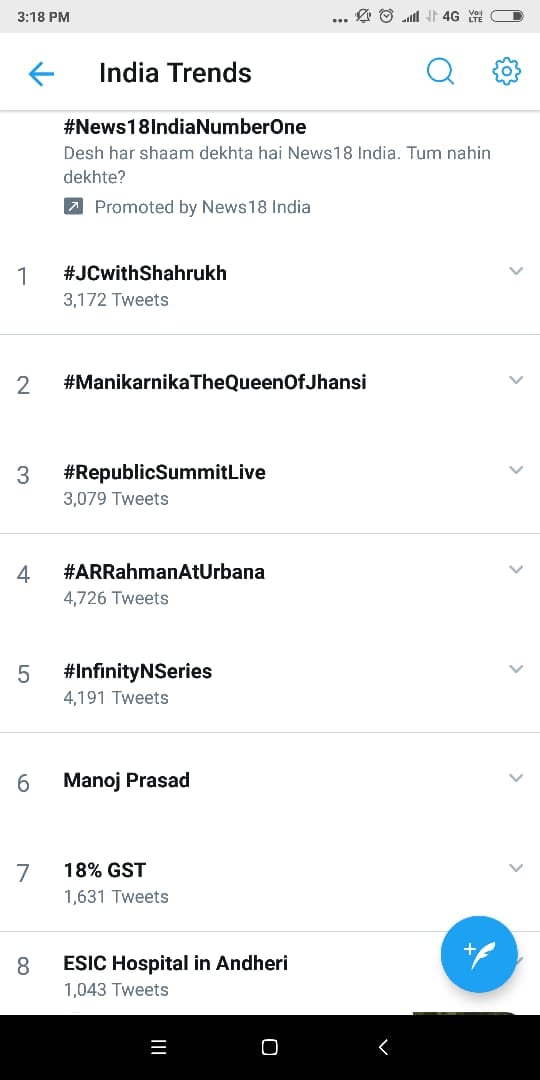A portrait-oriented image, seemingly captured from a cell phone, features a gray banner across the top. On the far left, the banner displays the time as 3:18 PM. Moving towards the center, there are three horizontal dots followed by icons indicating that the sound is off, an alarm clock, full cell phone service, 4G LTE connectivity, and a battery icon showing approximately 25% charge.

Below this banner, there is a blue arrow pointing to the left next to the text "India Trends." To its right, there are a blue search icon and a blue gear icon. A thin gray line separates this section from the next, which reads "#News18India Number One" followed by text in Hindi, and then "Number One" again, with a dropdown arrow on the right.

Further down, the text "JC with Sharmuka, 3172 tweets" is displayed, separated by another thin gray line from the next rankings, which list "#2" and "#3". Next to position two, it reads "#Manikarnika, The Queen of Jhansi."